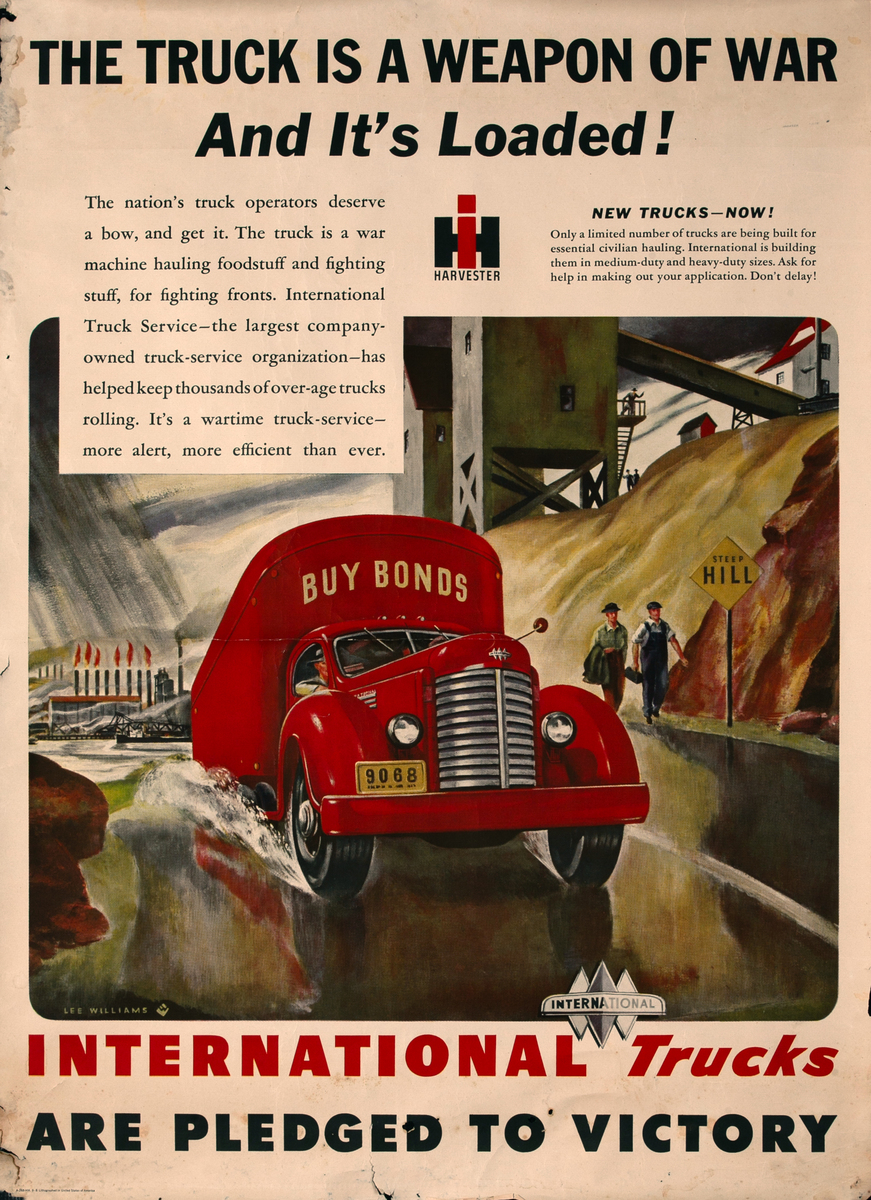The image is a digitized advertisement from the 1940s showcasing a red, medium-duty 'International' truck adorned with the slogan "Buy Bonds." At the top, bold black text proclaims, "The truck is a weapon of war and it's loaded." The truck, styled in a classic 1940s design with a noticeable front grille, highlights the essential role of trucks in wartime, emphasizing their necessity for civilian and military logistics. 

A detailed examination of the truck reveals it traveling down a street with notable features, including a soldier seated in the passenger seat, symbolizing its contribution to the war effort by transporting both foodstuffs and military supplies. The advertisement underscores that "International trucks are pledged to victory," with a reminder that only a limited number of trucks are currently being built for essential civilian hauling by International, available in medium-duty and heavy-duty sizes.

In the background, the street is flanked by a steep hill with buildings, and two pedestrians can be seen walking along the road. A sign at the bottom further reinforces the message: "International Truck Service, the largest company-owned truck service organization, has kept thousands of overage trucks rolling. Its wartime truck service is more alert, more efficient than ever." This advertisement appeals to the sense of urgency and patriotism of the time, encouraging quick action in securing these vital vehicles for the war effort.